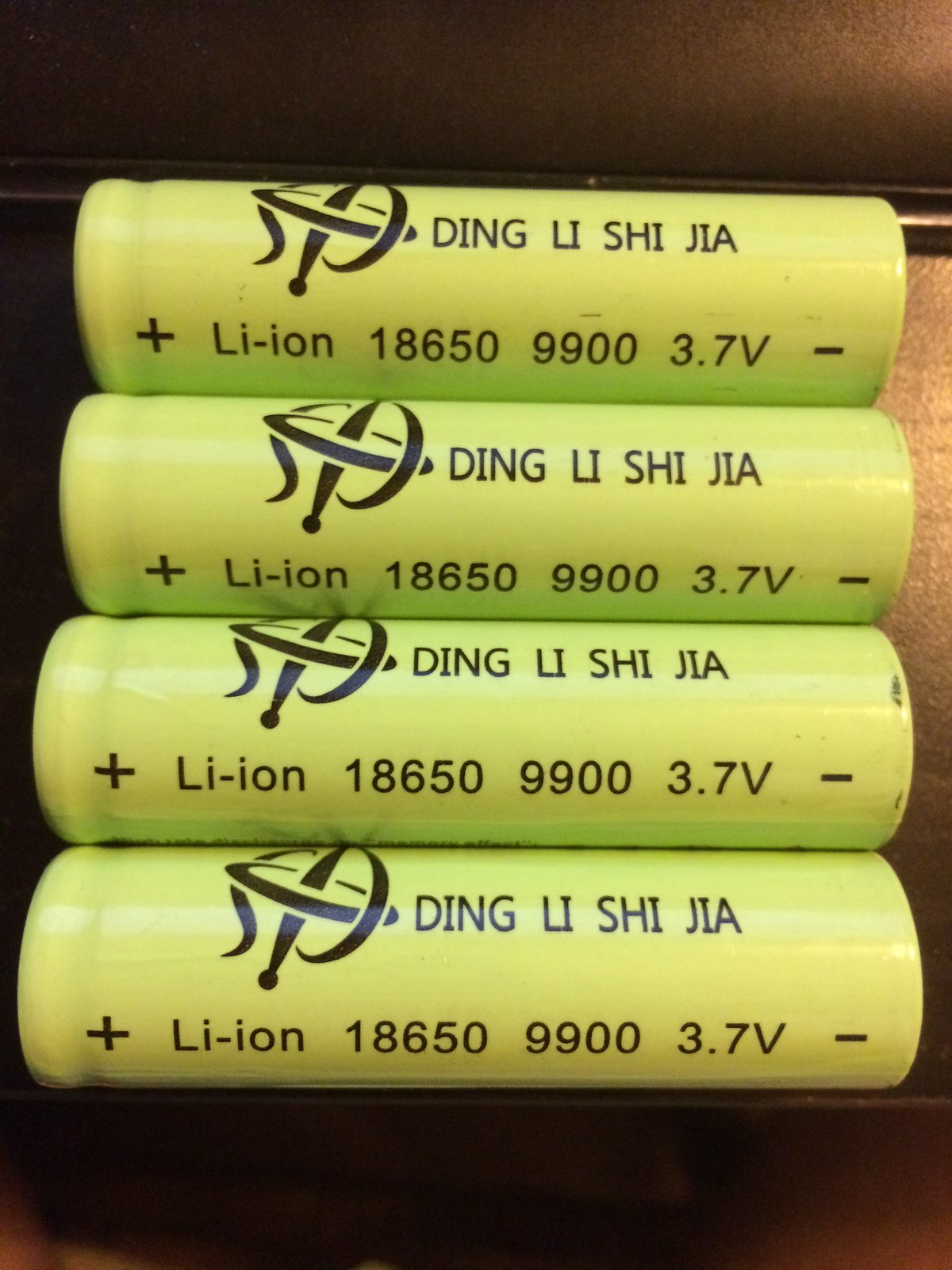This close-up photograph captures four yellow lithium-ion batteries, specifically labeled as 18650 9900 3.7V. The batteries are neatly stacked one on top of another on a dark brown wooden surface, which transitions to a lighter brown in the background, possibly a wall or a different part of the same surface. The batteries have a distinctive black design resembling a spinning top in the upper left corner, and beside it, the text “Ding Li Shi Jia” in black letters. Each battery clearly indicates the polarity with a plus sign (+) on the left side and a minus sign (-) on the right side. Additionally, they are uniformly labeled with "Li-ion 18650 9900 3.7V" below the logo.